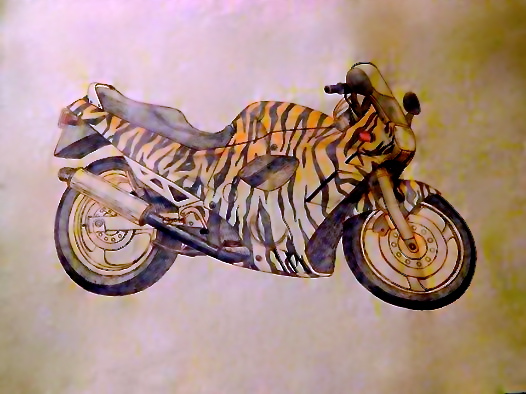This color photograph showcases an intricately detailed drawing of a motorcycle, which dominates the majority of the page. The motorcycle, facing right, is primarily black but features an eye-catching tiger stripe pattern in vivid orange and black along the right half of the saddle and beneath it, extending down to the spokes of the wheels. The background paper has a white base with a slight pinkish hue on the left, gradually transitioning to a greener tint towards the right and the bottom left corner. This variation could be due to discoloration or intentional coloring. The motorcycle is equipped with metallic handlebars on the right side and a metallic tube that runs through the left wheel, adding to the realism and detail of the artwork.